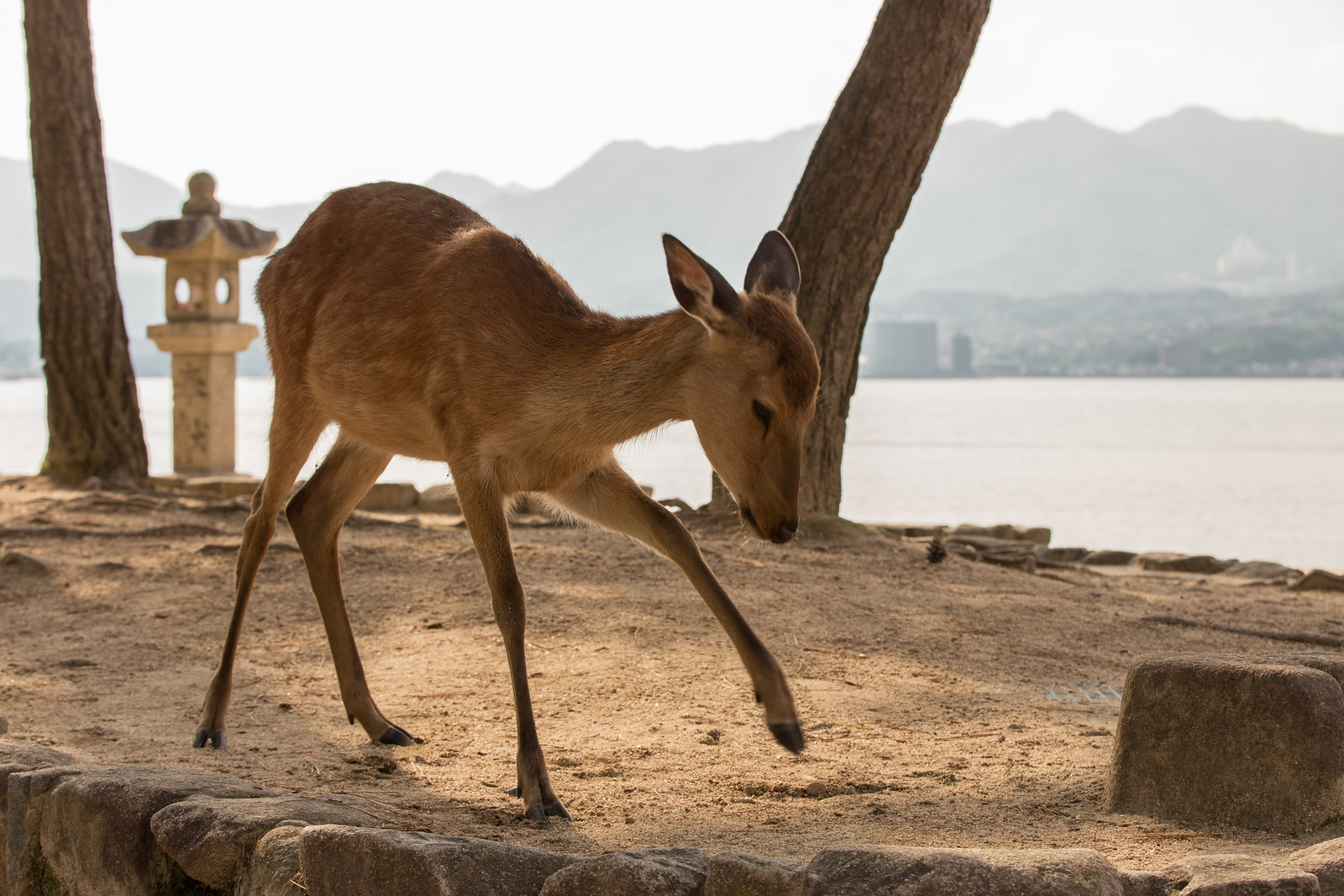A young deer, slightly older than a fawn as indicated by the absence of spots, is depicted facing to the right and standing on a broad expanse of sand. The deer, light brown with darker ears and a black nose, appears to be in the process of taking a step, with its head down and front left leg lifted. Immediately in front of it and slightly to the right lies a square rock. The sandy area it walks on is bordered by large, flat-topped rocks, resembling a low stone wall. In the background, two trees, one of which is leaning to the right, frame a vast body of water. Across the water, a distant shoreline with buildings can be seen, backed by a looming mountain range silhouetted against the horizon.